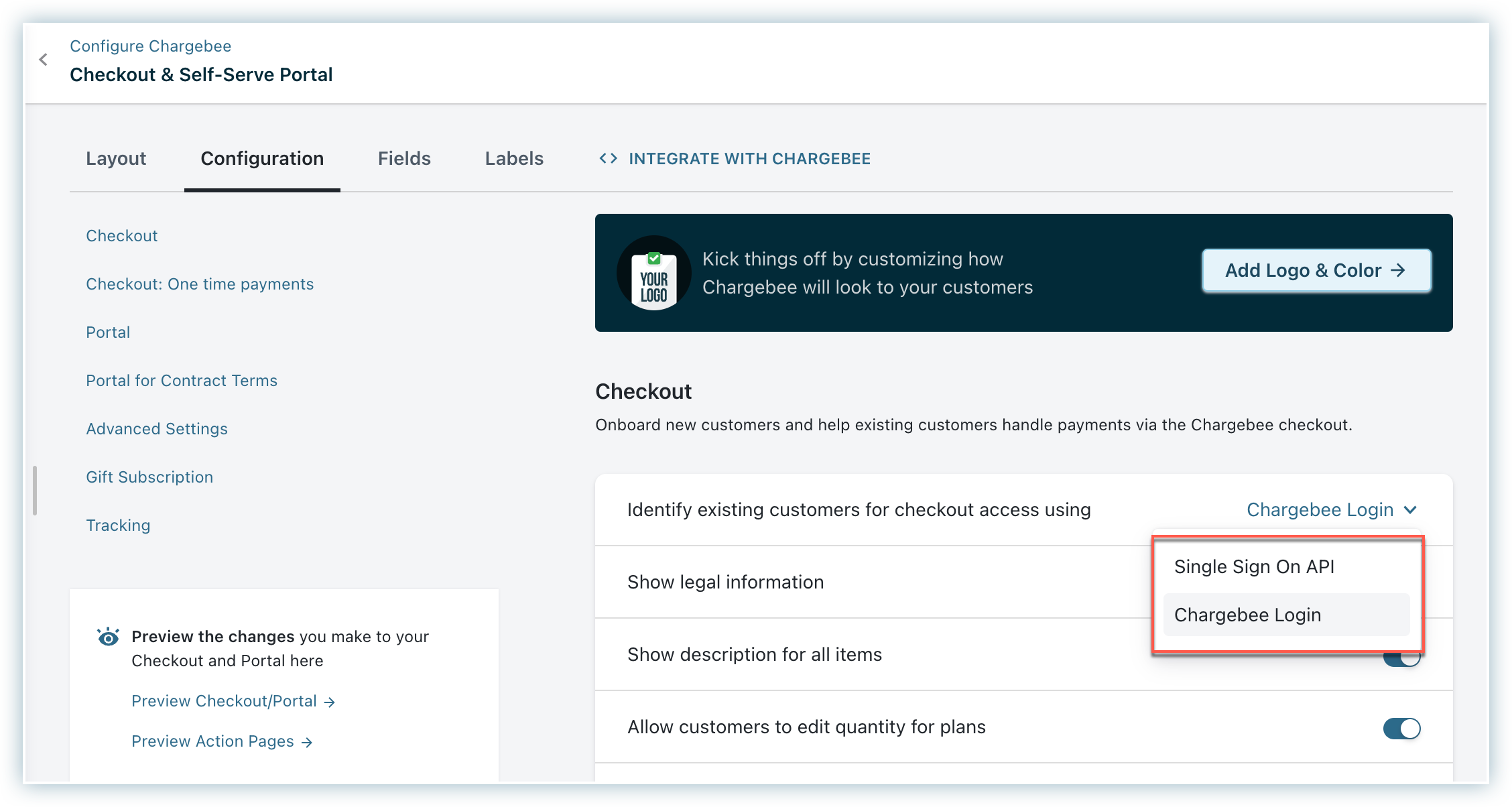This is a detailed screenshot of the ChargeBee configuration interface. The image is rectangular, featuring an upper left corner header in blue text that reads "Configure ChargeBee." Directly below, in bold black text, is the title "Checkout & Self-Serve Portal," accompanied to the left by a small black arrow pointing left, resembling a sideways "V."

The background is light gray. The upper-left section of the screen displays a menu with options arranged horizontally: "Layout," "Configuration" (bolded and underlined), "Fields," and "Labels." To the right of this menu are left and right blue arrows, also resembling sideways "V"s, with the blue text "Integrate with ChargeBee" beside them.

On the left side of the screen, there is a vertical menu listed in blue text: "Checkout," "Checkout: One-Time Payments," "Portal," "Portal for Contract Terms," "Advanced Settings," "Gift Subscription," and "Tracking." Beneath this menu is a white square housing a blue icon and bold text reading "Preview the Changes." Below this, in regular black text, it says, "you make to your checkout and portal here." A clickable blue link labeled "Preview Checkout / Portal" is situated below this text, followed by another link titled "Preview Action Pages."

On the right side of the screen at the top, there is a dark rectangular area labeled "Kick Things Off" with accompanying text: "By customizing how ChargeBee will look to your customers." Adjacent to this is a rectangular button labeled "Add Logo and Color."

Below this section is a white box for "Checkout" settings. Inside this box is a bulleted list with options: "Identify Existing Customers for Checkout Access Using," "Show Legal Information," "Show Description for All Items," and "Allow Customers to Edit Quantity for Plans." Additionally, on the right side of this box are two lines of text, "Single Sign-on API" and "ChargeBee Login," each outlined with a red rectangle.